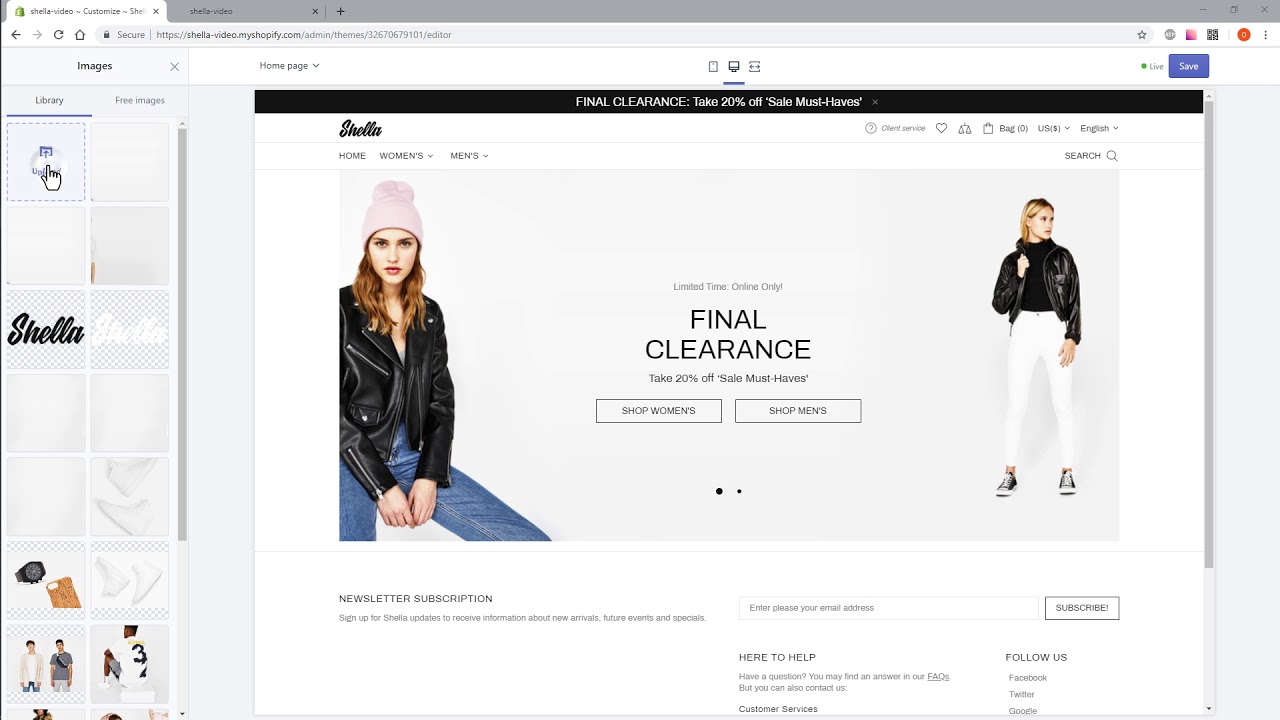The image is a screenshot of a web browser displaying a fashion retailer's website, identified as either "Shella" or "Sheila." The webpage is showcasing a final clearance sale, prominently featuring a large promotional image. In the image, there is a young woman wearing a budget-friendly looking motorcycle leather jacket paired with a pink beanie. Standing to her right is another woman dressed in white pants and similar casual apparel. The overall aesthetic suggests a fast fashion brand, presenting clothing that appears uninspiring and indistinct, common to many such brands. The website's design is also noted to be generic and unoriginal, blending into the multitude of similar fashion e-commerce sites. The pricing of the items on sale is ambiguous, potentially ranging from inexpensive to surprisingly high, adding to the uncertainty and uniformity of the brand's presentation.